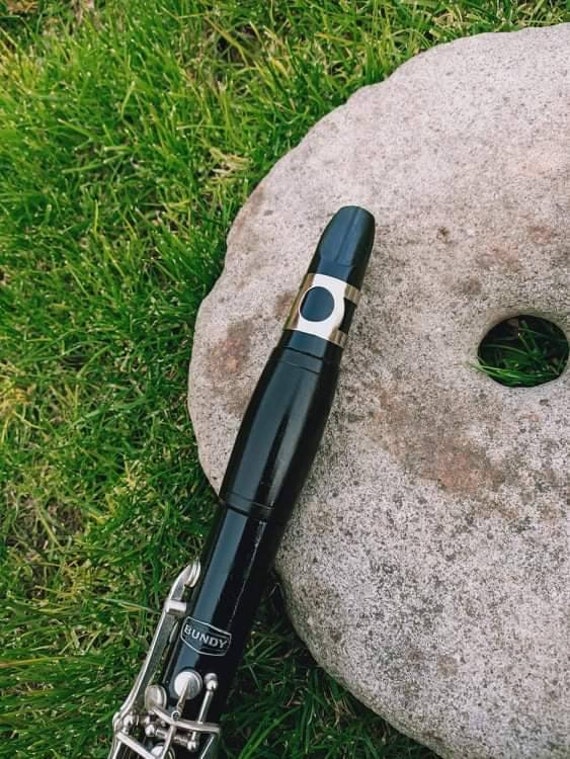A black clarinet is prominently featured in this outdoor photograph, elegantly leaning against a circular, beige stone that rests on vibrant green grass. The instrument exhibits striking silver buttons and dials along its body, used to play its various notes. Near the top of the clarinet, a silver ring encircles the mouthpiece area, adding to its refined appearance. The name "Bundy" is clearly visible in white lettering on the instrument. The stone itself is unique, characterized by a circular hole in its center through which grass can be seen. The composition presents a beautiful contrast between the clarinet’s sleek black and silver features, the beige hues of the stone, and the lush greenery that surrounds them.